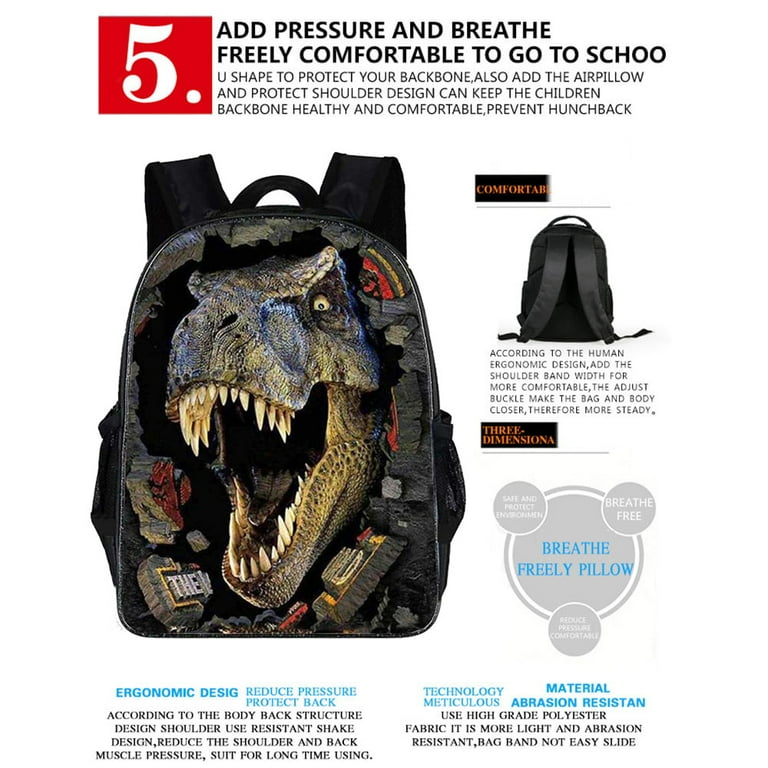This advertisement displays a black backpack featuring a lifelike T-Rex design with sharp teeth and yellow eyes, seemingly coming out of the backpack for a striking 3D effect. Positioned against a white background, the backpack bears the number 5 in white within a red box at the top left. The title above the backpack reads, "Add Pressure and Breathe Freely, Comfortably to Go to School." Detailed descriptions highlight its ergonomic U-shape design to protect the backbone, an air pillow, and shoulder protection features aimed at maintaining a child's healthy posture and preventing hunchback. Comfortable shoulder bands can be adjusted for a closer fit, ensuring stability. Additional features include abrasion-resistant, high-grade USA polyester fabric, which is light and prevents the bag from easily sliding. Further annotations emphasize its human ergonomic design, reducing shoulder and back muscle pressure, making it suitable for long-term use. The advertisement also includes the phrases "Breathe Freely Pillow" and highlights "Three-Dimensional" and "Ergonomic Design, Reduce Pressure, Protect Back" in varying text colors to spotlight the backpack's focus on comfort and durability.